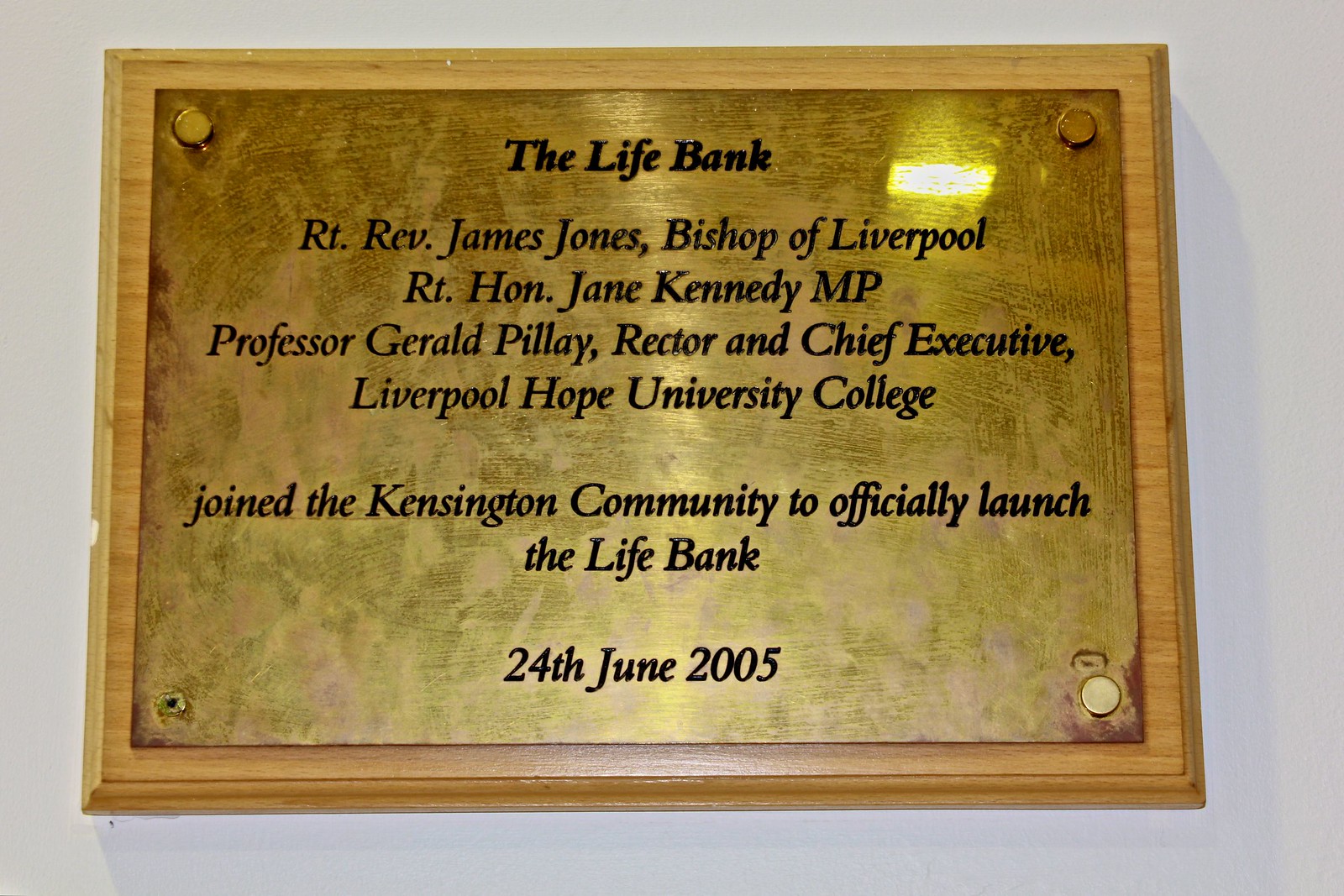This photograph captures a rectangular wooden plaque with a golden metal plate affixed to it. The light tan wood creates a distinct border around the landscape-oriented plaque. The metal plate, which has a golden hue, is attached to the wood by three golden bolts: one at the top right corner, one at the top left corner, and one at the bottom right corner, with the bolt in the bottom left corner conspicuously missing. Engraved in black letters on the metal plate is the following text: "The Life Bank, R.T. Reverend James Jones, Bishop of Liverpool, R.T. Honorary Jane Kennedy, M.P., Professor Gerald Pillay, Rector and Chief Executive, Liverpool Hope University College. Joined the Kensington community to officially launch The Life Bank, 24th June 2005." The plaque appears to be either hanging on a white or light gray wall or laid on a white surface, and there is a noticeable reflection of light at the top right corner of the plaque.